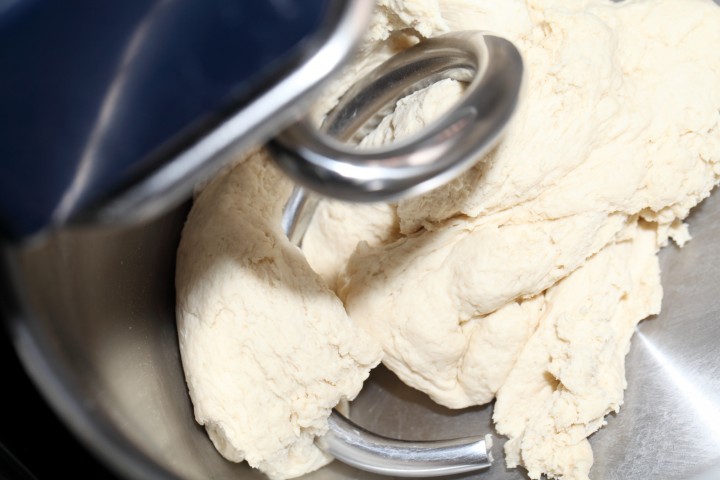The image is a clear, extreme close-up of a stainless steel KitchenAid mixer in action, prominently featuring its spiral kneading attachment entangled with a pale, light-colored clump of dough. The mixer, decorated with dark blue and metallic trim, has its distinct corkscrew-like attachment descending from the upper left to the dough at the bottom center, visibly working to shape the dough into a ball. The scene is well-lit, showcasing the folds and texture of the dough within the sleek, reflective surface of the aluminum bowl. The overall setting and image clarity are high, with no text or additional elements in the frame.